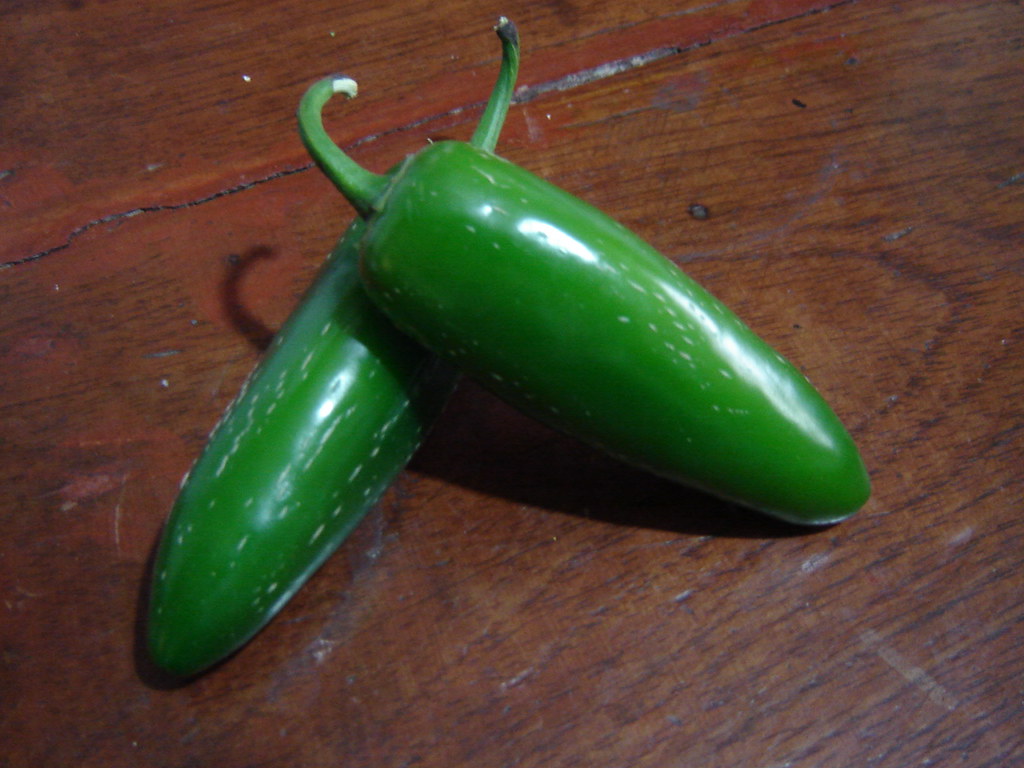In this detailed image, two green jalapeno peppers rest on a brown wooden surface with a prominent wood grain pattern, possibly an older table bearing a few cracks and stains. The jalapenos, which appear to be miniature due to their small size, have smooth, glossy, and shiny skins. Each pepper features distinctive markings: one has white streaks at its end while the other displays a darkened tip. Both chilies have short, curled stems, giving them a hook-like appearance. The peppers are positioned to form a triangular shape, with one lying on its side and the other propped up against it, creating a harmonious composition. Light reflects off their surfaces, highlighting their ripe and well-cared-for condition. Overall, the scene exudes a rustic charm, accentuated by subtle brown marks on the jalapenos and the aged, stained look of the wooden table beneath them.